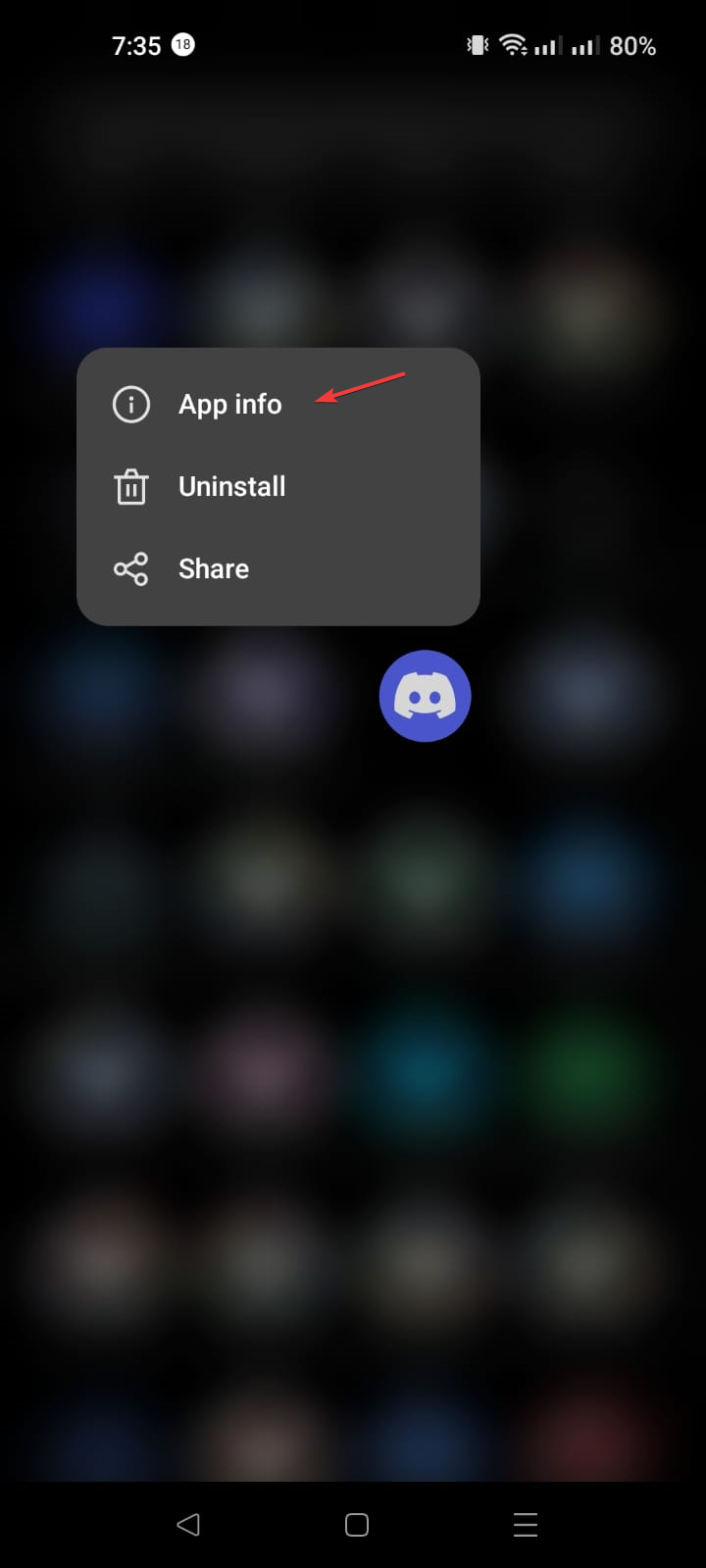The image is a detailed screenshot captured from a cell phone screen. At the top part of the screen, there is a black border displaying the time "7:35" in white text. Additionally, there is a circular icon with a white background containing the text "1E." Following this, various system icons are visible, including the cell phone vibrate icon, Wi-Fi signal indicator, and a small up and down arrow representing data transfer. There are also two cell phone signal bars and a battery indicator showing an 80% charge.

Below these icons, a pop-up notification appears, characterized by its dark charcoal gray or light black background. This pop-up features a circle with the letter "i" inside it, indicating information. Next to this symbol, the text "App Info" is displayed, starting with a capital "A." There is also an arrow pointing diagonally right towards the "App Info" text.

Underneath this text, there are three options: 
1. An icon of a garbage can accompanied by the text "Uninstall" with a capital "U."
2. A share button labeled "Share" with a capital "S."
3. Below the gray square box, there's a small blue-violet circular icon that appears to depict a remote control.

At the bottom of the screen, the navigation bar is shown, containing three icons: a left-pointing arrow, a square, and three vertical lines, representing the back, home, and recent apps functions, respectively.